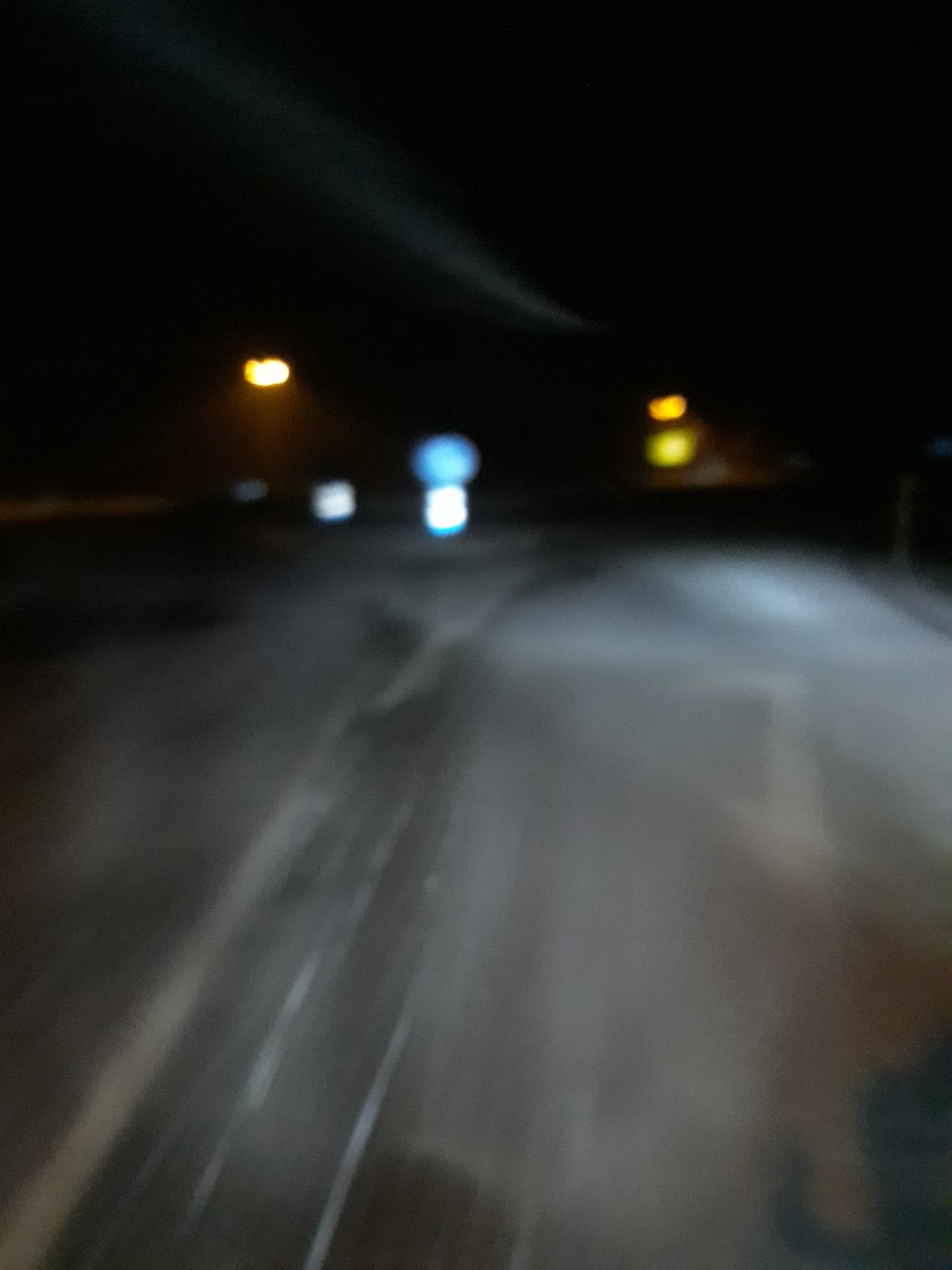This is a very blurry nighttime photograph ostensibly taken from a moving vehicle, possibly a car or an airplane. The photo features a dark, pitch-black sky with streaks of light that may suggest movement. The ground appears to be a roadway with pavement visible below, displaying faint white lines that may be road markings or thin lines on a runway.

There are multiple light sources in the image, situated in various positions. On the left side, the lights are orange and white, while the center lights are blue and white, and the right side showcases orange and yellow lights. These lights could potentially be the rear lights of vehicles or illumination from other sources like street lamps or runway lights. A faint white streak extends from the top left corner towards the center, possibly indicating the motion of an airplane or a cloud formation.

In the middle of the photograph, there appear to be some signs or indicators, including a white sign on the middle-left side and a blue sign in the center. The pavement below reflects a white-ish, gray-ish hue, which might suggest snow-covered ground. In the bottom right corner, there's a vague shadow that might be a person holding up a cell phone, though it's difficult to discern due to the image's blurriness. Overall, the photograph captures a scene set at night, characterized by indistinct lights and movement.